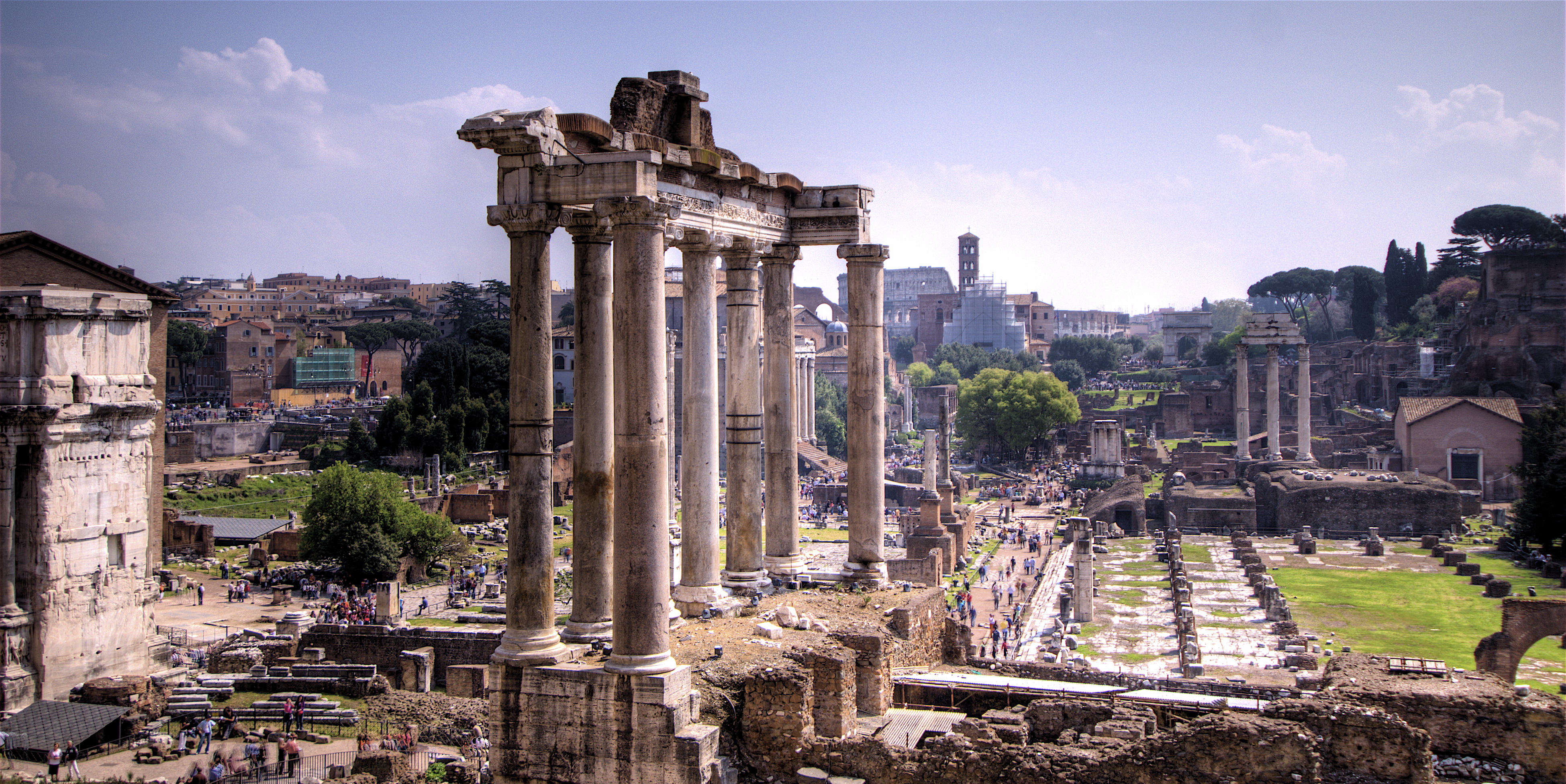The color photograph captures a stunning juxtaposition of ancient ruins set against a modern cityscape. Centered prominently in the image is an ancient Roman or Greek structure, characterized by its iconic columns and scattered architectural fragments. The ruins are set on a mountainous terrain, dotted with green trees, grass, and shrubbery, contributing to the historical ambiance of the scene.

Numerous people are seen exploring and congregating throughout the ruins, from the left to the right of the photograph, enhancing the sense of scale and activity. To the far left, a white stone building stands out amid the ancient landscape. The middle of the image features a tall, columned tower, surrounded by other ancient edifices in varying states of decay. Patchy grassy areas and stone objects are scattered around, adding to the texture of the scene.

In the backdrop, a modern city emerges, with a variety of buildings capped under a cloudy, light blue sky. The sky, devoid of the sun, features scattered white clouds, adding to the atmospheric depth of the photograph. Despite the mix of historical and contemporary elements, the image maintains a harmonious blend of browns, creams, grays, and greens, punctuated by the subtle blues of the sky and a small blue-gray lake. The photograph, taken from a considerable height and distance, provides a comprehensive view of this rich, multi-layered landscape.